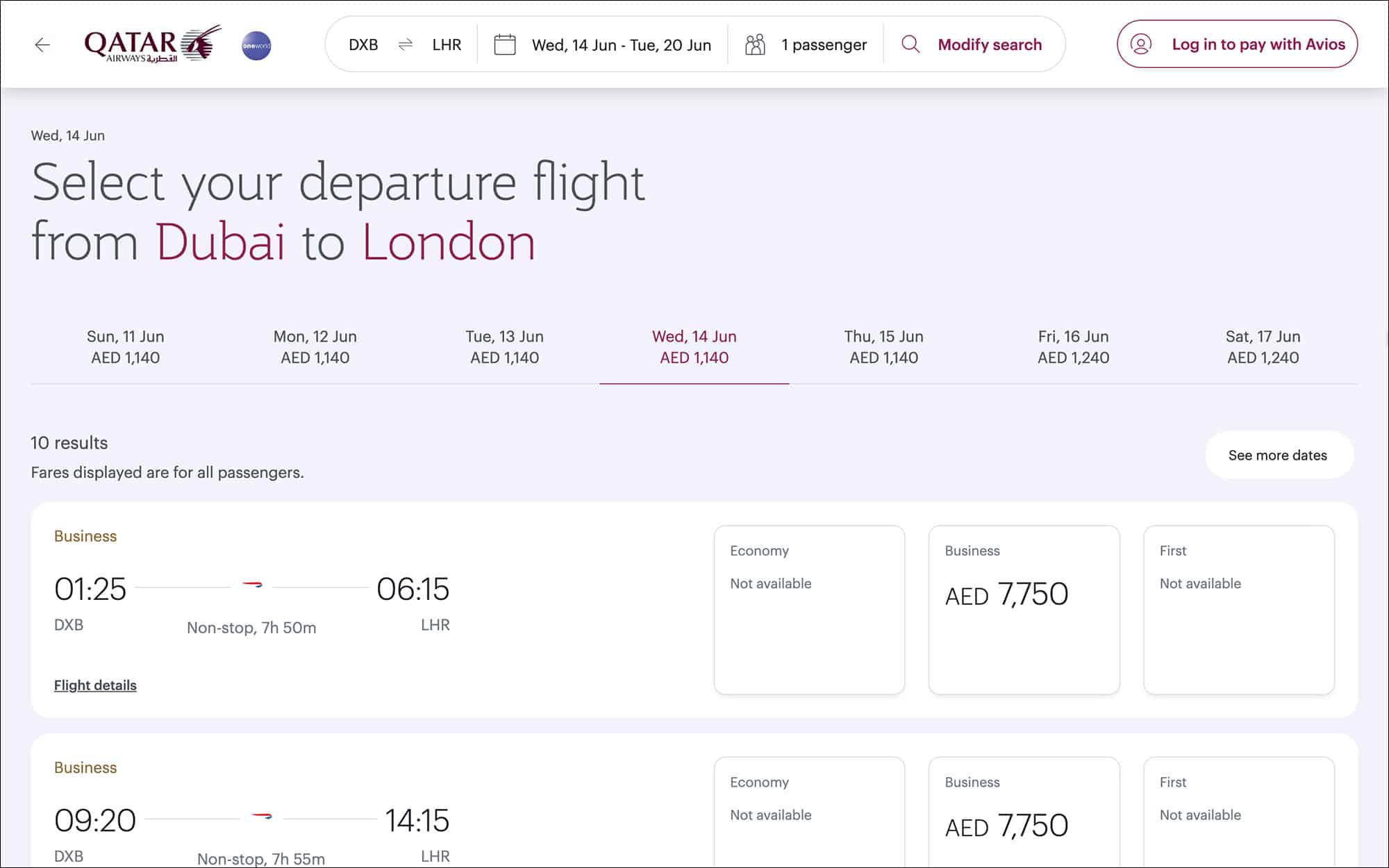The image depicts a person navigating the flight booking section of the Qatar Airways website. The visible interface shows the user is trying to book a flight from Dubai (DXB) to London (LHR), with the intended travel dates from Wednesday, 14th June to Tuesday, 20th June. The page clearly indicates it is for one passenger and includes options to modify the search or log in to pay with Avios points.

At the top of the page, the Qatar Airways logo is prominently displayed in the upper left corner. The travel route (DXB to LHR) and the travel dates are listed horizontally. Below that, instructions prompt the user to select their departure flight from Dubai to London on Wednesday, 14th June. A list of dates and corresponding fares is provided: 

- Sunday, 11th June: AED 1140
- Monday, 12th June: AED 1140
- Tuesday, 13th June: AED 1140
- **Wednesday, 14th June: AED 1140 (highlighted in purple)**
- Thursday, 15th June: AED 1140
- Friday, 16th June: AED 1240
- Saturday, 17th June: AED 1240

For the selected date (Wednesday, 14th June), it states "10 results available," specifying that the fares are displayed for all passengers. The available flights and fares are then detailed as follows:

1. Business Class flight leaving at 12:25 PM, non-stop, with a flight duration of 7 hours and 50 minutes, arriving at 6:15 PM at LHR. Economy class is not available, and the Business class fare is AED 7750. First class is also unavailable.
   
2. Business Class flight departing at 9:20 AM, non-stop, with a flight duration of 7 hours and 55 minutes, arriving at 2:15 PM at LHR. Economy class is not available, and the Business class fare is AED 7750. First class is also unavailable.

The rest of the screen contains no additional text or information, emphasizing the user's current task of booking a flight from Dubai to London.